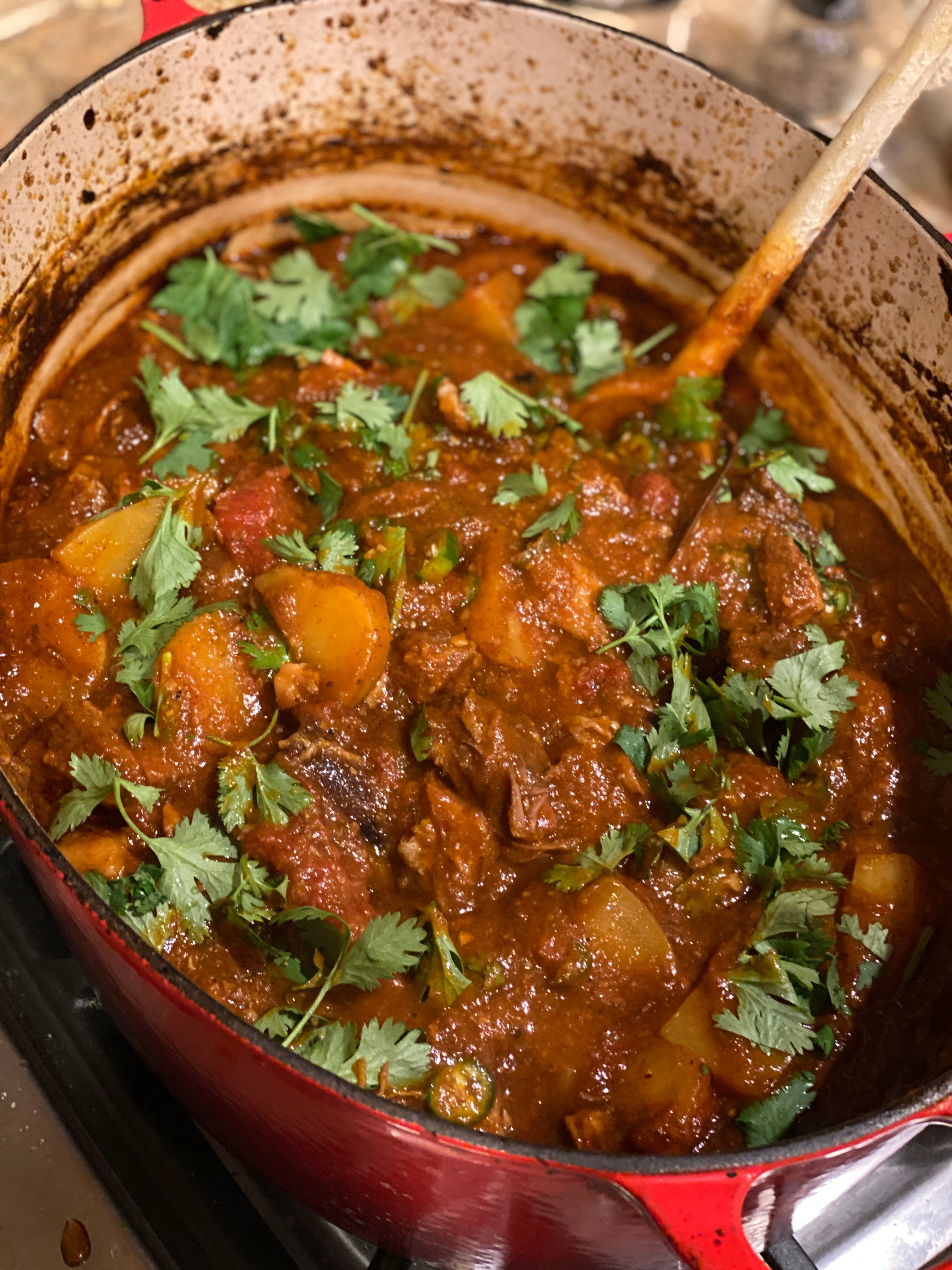This overhead close-up photograph captures a hearty stew simmering in a red, oval-shaped cast iron pot, set on a stove. The pot's white interior is brimming with a thick, brown gravy enveloping chunks of stew meat, potatoes, and carrots. A large wooden spoon extends from the pot, ready for stirring. The stew is garnished with a generous sprinkle of finely chopped greenery, likely cilantro or parsley, adding a pop of color to its rich browns, light oranges, and reds. The crusty edges along the pot and the visible texture of the countertop below suggest the photo is primed for a recipe site or culinary showcase. No people or text are present, ensuring full focus remains on the mouth-watering meal.